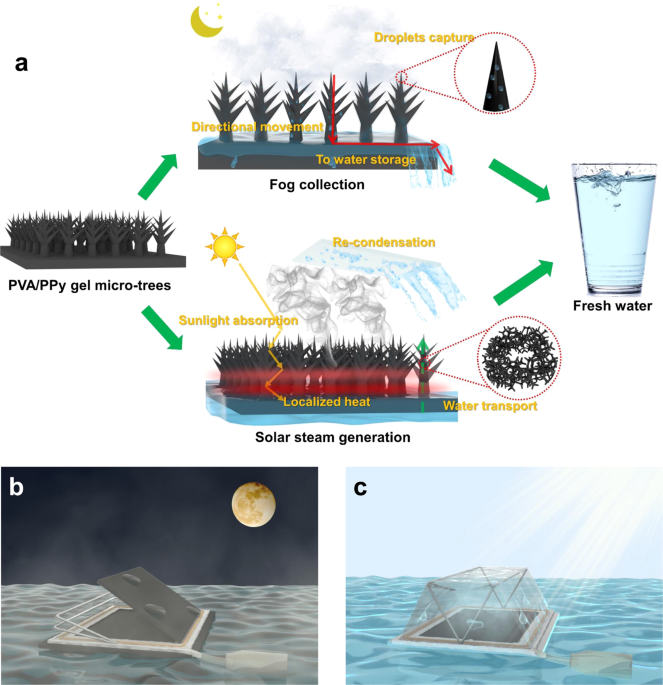This infographic, set against a plain white background, showcases the process of water condensation and solar steam generation in a visually detailed and segmented manner. The graphic is roughly square in shape, measuring between 5 to 6 inches each side, and is divided into an upper half and a lower half.

In the upper half, the main image, labeled "A" in the top left corner, is a comprehensive flowchart detailing the water collection process. It centers on a digital representation of "PVA, PPY, Gel Microtrees." These spiky, tree-like structures rooted in ground and water are integral to fog collection and water transport mechanisms. Above these trees, the chart depicts a moon and clouds, highlighting the concept of fog collection through directional movement towards water storage. Downward arrows illustrate how water droplets are captured and directed towards a glass of fresh water. The flowchart also outlines a daytime process involving the sun, showcasing steps like recondensation, sunlight absorption, and solar steam generation, again culminating in the collection of fresh water.

Below this main graphic, two images labeled "B" and "C" illustrate the operation of a floating device within different environmental contexts. Image "B" features a 3D model of this device at night, floating on water under a dark, moonlit sky. Image "C" presents the same model during the day with a blue sky and sunlight, now covered by a clear plastic hatch that captures condensation, showing the transformation from night to day and the device's operational dynamics.

Emphasizing renewable processes, this infographic clearly outlines a sustainable method for converting fog and sunlight into fresh, potable water.